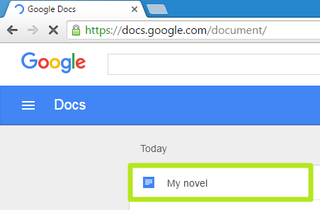At the top of the image, a blue background features an open browser tab displaying "Google Docs" in black text, with the first letter of each word capitalized. To the right, there is a black X for closing the tab. Adjacent to the tab is a light blue parallelogram, whose purpose is unclear.

Below this, on the next row to the left, there is a dark grey arrow pointing left, followed by a light grey arrow pointing right. Next to these arrows is a dark grey X, indicating a web browser tab. The browser bar itself is white, featuring a green lock icon and the text "HTTPS" in green, followed by "://docs.google.com" in black text, then "/document/" in grey; the browser content is zoomed in too much to see any further.

Beneath this, the background changes to white, displaying the colorful Google logo: a capital blue G, followed by a red O, a yellow O, a lowercase blue G, a lowercase green L, and a lowercase red E. Below the logo is a search box, also zoomed in too much to see its end, featuring a white interior with a grey border.

A blue banner stretches across beneath the search box, adorned with three white lines and the word "Docs" in white, capitalized letters. The background transitions to light grey, displaying the word "Today" in black. Underneath this, there is a rectangular box with a green border and a white interior, containing the text "My Novel" in black.